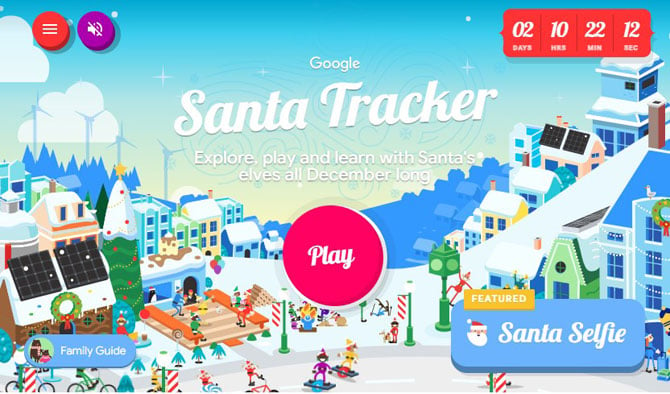A whimsical, rectangular cartoon illustration features an enchanting winter town scene. The vibrant, snow-covered landscape is adorned with festive elements that evoke the magical spirit of Christmas. Notably, a towering outdoor Christmas tree, decorated with a shining star, red baubles, and a dusting of snow, stands prominently amidst candy cane flags and bustling elves.

Centrally placed text reads "Google" in small lettering, while "Santa Tracker" is boldly displayed in large, eye-catching font. Below this, an invitation to "Explore, play and learn with Santa's elves all December long" is written in crisp white.

Dominating the bottom of the image, a large red circle with the word "Play" inscribed in white beckons viewers to engage. In the upper right corner, a red background displays a countdown in white font: "02 days 10 hours 22 minutes and 12 seconds" until Christmas. Additionally, in the bottom right corner, a blue section highlights "Featured: Santa Selfie" with a charming headshot of Santa Claus, showcasing his familiar red hat, white beard, and simple, expressive features.